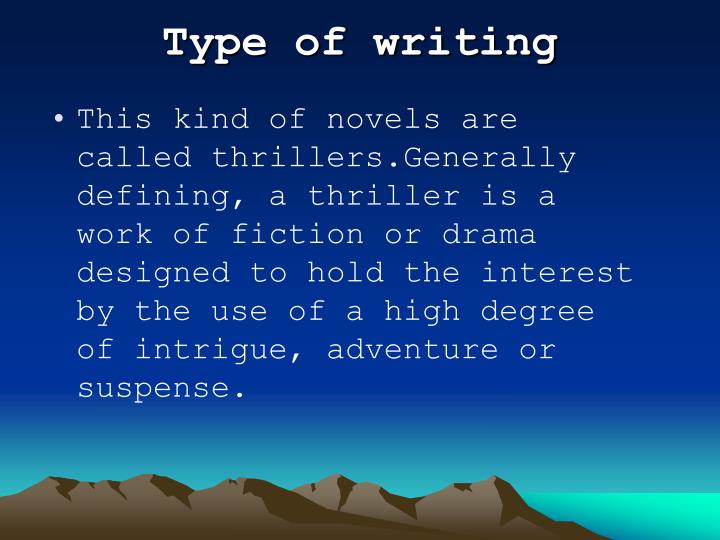This instructional slide features a prominently bold title in white Courier font at the top center, stating "Types of Writing." Beneath it, there is a single bullet point that reads: "This kind of novels are called thrillers. Generally defining, a thriller is a work of fiction or drama designed to hold the interest by the use of a high degree of intrigue, adventure, or suspense."

The background is a simple yet detailed illustration of nature. The sky, taking up most of the slide, transitions from dark blue at the top to a lighter blue or teal as it descends. Below the gradient sky, at the very bottom of the slide, lies a minimalistic depiction of a mountain range. The mountains, portrayed in lighter brown with darker brown shadows, occupy only a small portion of the slide. Behind the mountains lies an ocean, characterized by an aqua gradient blending into a darker blue. The overall visual theme is nature-inspired, with a clear, illustrative style rather than photographic realism.